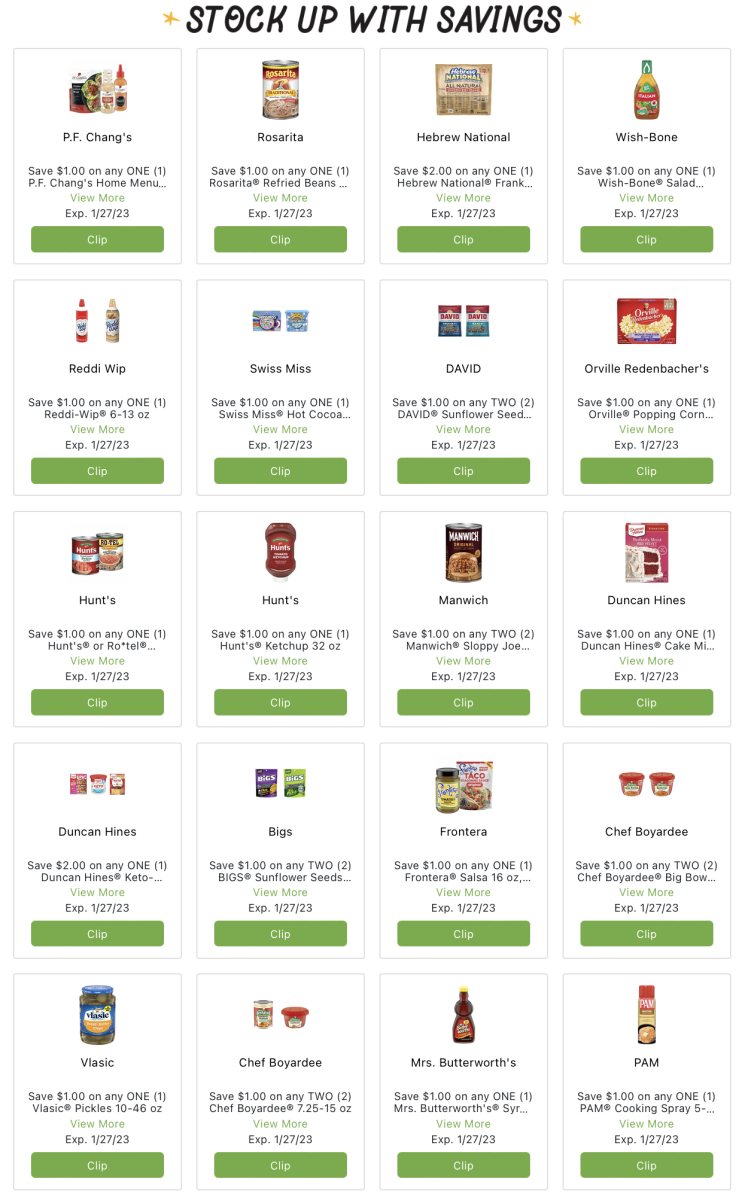The image showcases a vibrant green themed shot set against a stark white background, emphasizing an assortment of grocery items prominently stacked up in tiers. The display includes a variety of well-recognized brands and products aimed at highlighting savings. Among these are Shayne's Ramiro, Hebrew National sausages, Wish-Bone salad dressings, Ready Whip whipped cream, Swiss Miss hot chocolate, and David sunflower seeds. The display also features Bopper's snacks and multiple Hunt's products including a meatloaf sauce and a traditional ketchup.

Additionally, the image presents boxes of Duncan Hines baking goods: a cake mix and three different types of frosting. There are approximately six small containers from Chef Boyardee, with the first set consisting of microwaveable half cans and the second set comprising regular full-size cans alongside more microwaveable half cans. The arrangement skillfully combines various packaged foods, ranging from meal components to baking essentials, showcasing both their variety and their potential for significant savings.